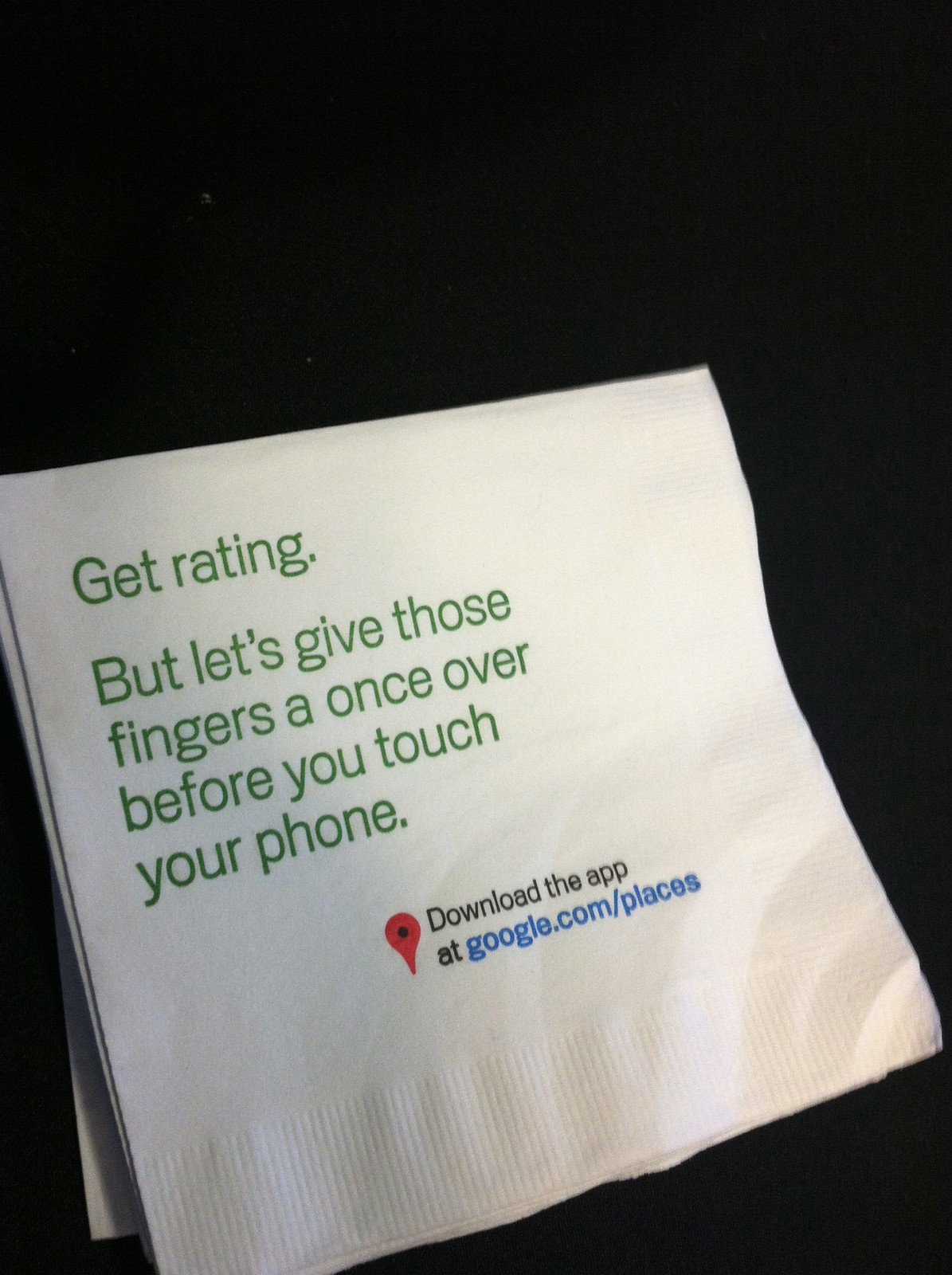The image features a white napkin set against a solid black background, angled slightly backward. Dominating the top left quarter of the napkin is bold green text which reads, "Get Rating, but let's give those fingers a once over before you touch your phone." Below this main message, at the bottom of the napkin, there is a prompt in black and blue text that says, "Download the app at google.com/places." To the left of this text is a small red Google Maps pin with a black center. The napkin appears to be part of a stack, likely used in a restaurant to encourage customers to rate their experience and download an app.